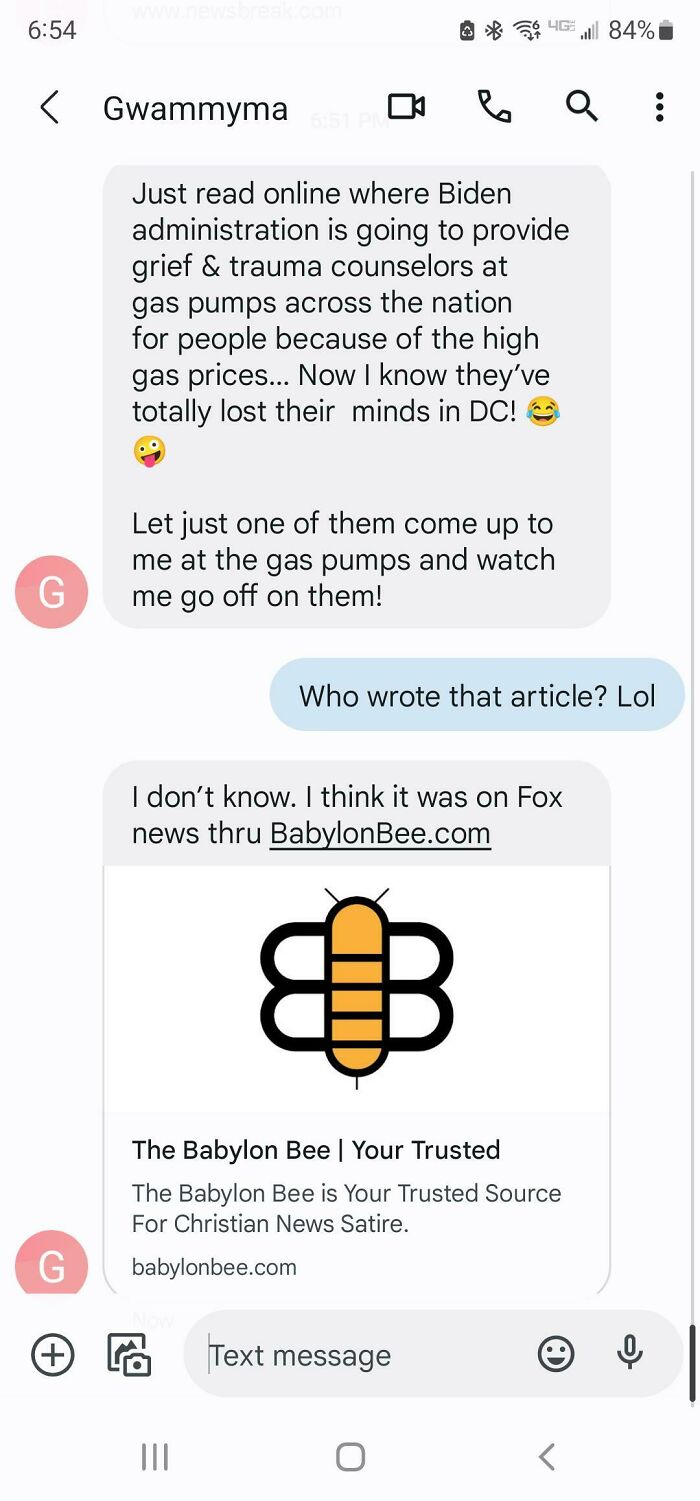Here's a detailed and cleaned-up caption for the screenshot of the phone:

---
*The screenshot shows the main screen of a smartphone. In the top-left corner, the time is displayed in black as "6:54", with the battery level at "84%". Below, there’s a left-pointing arrow icon next to the contact's name, "Gwammya". To the right of the name, several icons are visible, including a camera (indicating video call capability), a phone (for calling), and a magnifying glass representing search functionality. 

The conversation on the screen begins with a message from the contact, identified by a pink circle with a white "G" on a gray background. The text reads, "Just read online where the administration is going to provide grief and trauma counselors at gas pumps across the nation for people because of the high gas prices now. I know they lost their minds in DC," followed by a laughing emoji and a silly face emoji.

The recipient responds in black text, asking, "Who wrote the article?" The contact replies, "I don't know. I think it was on Fox News, Babylon Bee.com."

At the bottom of the screenshot, there is a promotional banner for The Babylon Bee. It has a white background with a black and yellow bee logo in the center. The text reads, "The Babylon Bee - Your trusted source for Christian news satire. BabylonBee.com."*
---

This caption provides a clear and comprehensive description of the content and layout of the screenshot.